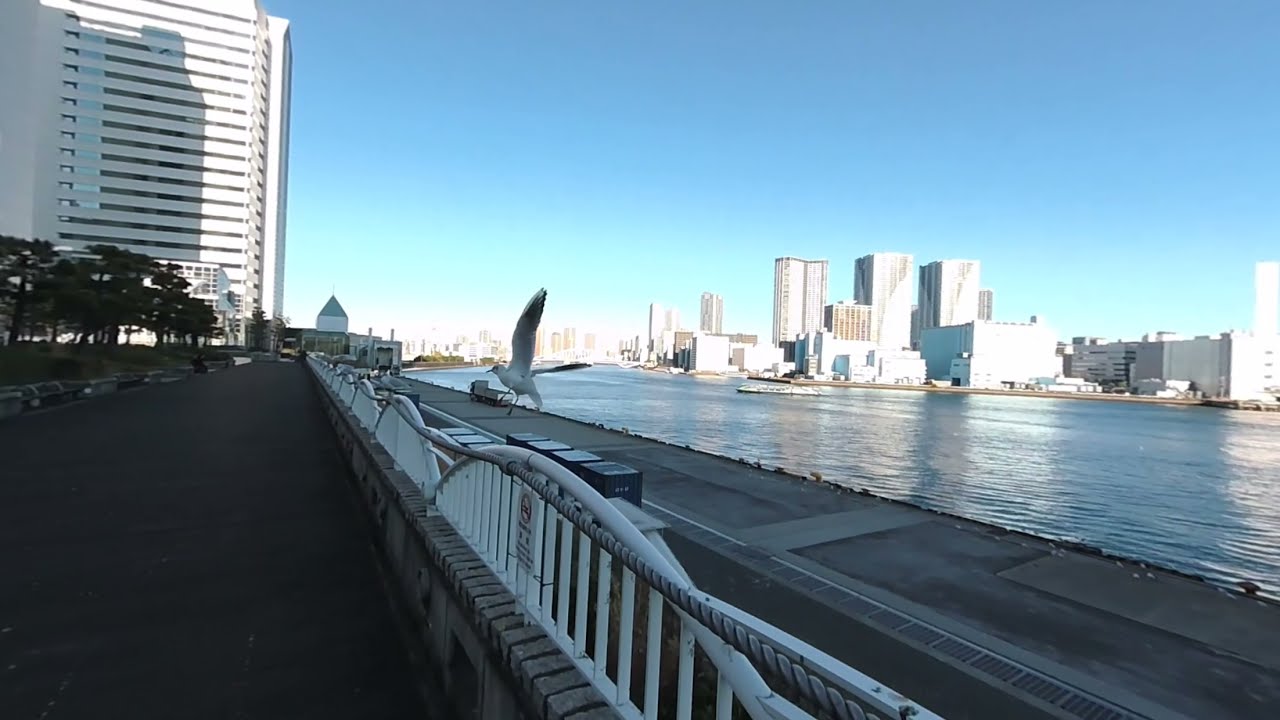The image captures a vibrant, sunlit scene of a modern metropolitan cityscape surrounding a tranquil blue body of water, likely a river or harbor. Taken from a pier, a white guardrail aligns the left-hand side, offering a vantage point of the scene. Immediately noticeable is a seagull prominently flying in the center of the image. The left side features small trees and a large white building, possibly a hotel or apartment complex, towering above surrounding structures. The right side showcases a flat cement dock lining the water, highlighting a mix of tall skyscrapers and mid-size buildings stretching into the horizon. The clear blue sky and bright sunlight enhance the vivid colors and sharp details, capturing an image devoid of people but filled with architectural and natural beauty.